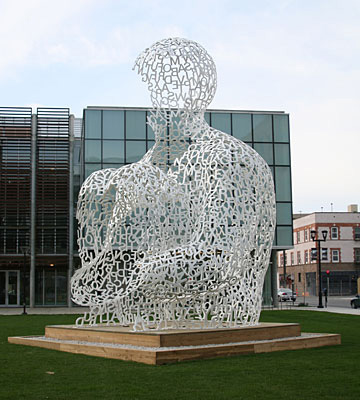The photo captures an outdoor art display situated on a plush, green grass field. Central to the image is a striking sculpture positioned atop two rectangular platforms, the lower one slightly larger than the one above. The sculpture itself is a see-through, white lattice configuration composed of interwoven alphabet letters, creatively forming the upper torso of a human figure. Though strikingly detailed, the figure is incomplete: the head is partially open with a noticeable void where the face should be, the neck connects only on one side, and the arms are truncated at the elbows with only one extending downwards.

In the backdrop, a modern building with an expanse of green glass windows rises four to five stories high. Adjacent to this is a smaller, three-story building in brown and tan, contributing to the urban setting. Street signs, a street light, and a passing car add to the city atmosphere. The sky above is clear and blue, further accentuating the vivid details of both the sculpture and its surroundings.